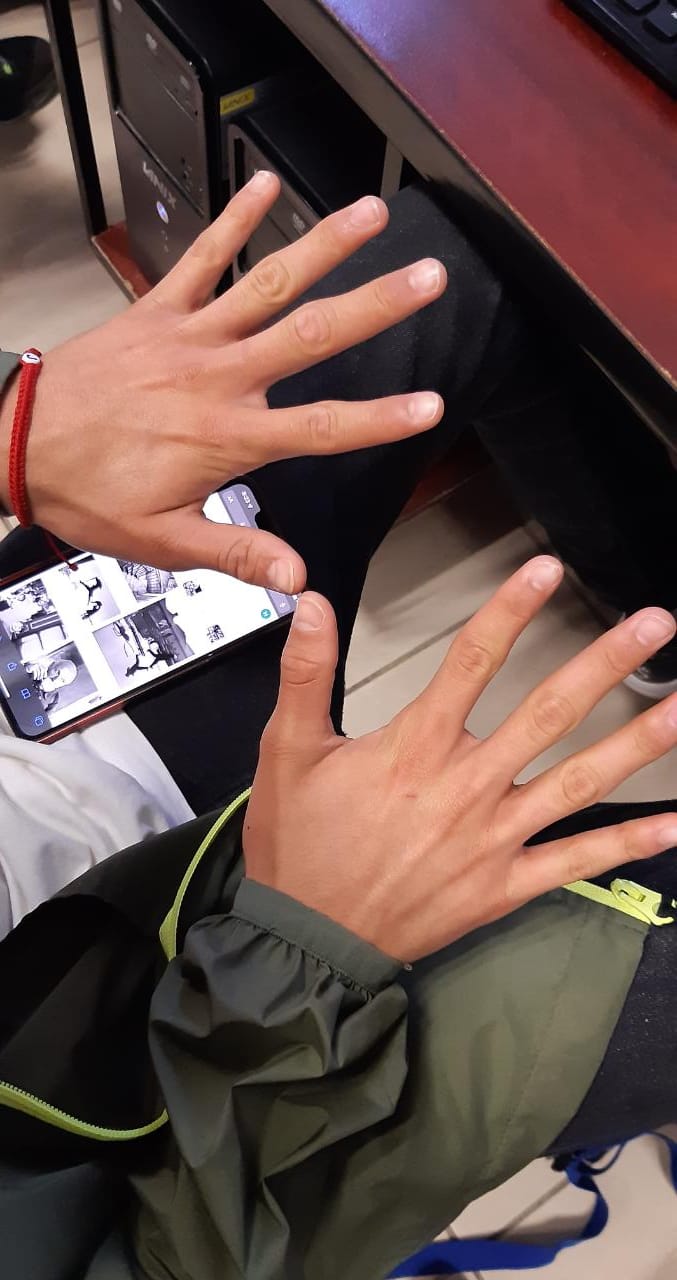The image shows a person, likely male, seated at a dark mahogany-colored laminated computer desk. He is wearing a green spring jacket with a yellow zipper, black jeans, and a white T-shirt. Only the tops of his thighs and his hands are visible. His hands are spread out in front of him in a manner reminiscent of showing off a new manicure, with thumbs pressed together, revealing nicely trimmed nails. A red bracelet adorns his left wrist. On his lap rests a mobile phone displaying a website with black and white photography. Beneath the desk, a couple of old-school tower computers are visible. The floor in the scene is light beige and tiled. Just a bit of the keyboard peeks in from the top right corner of the desk.